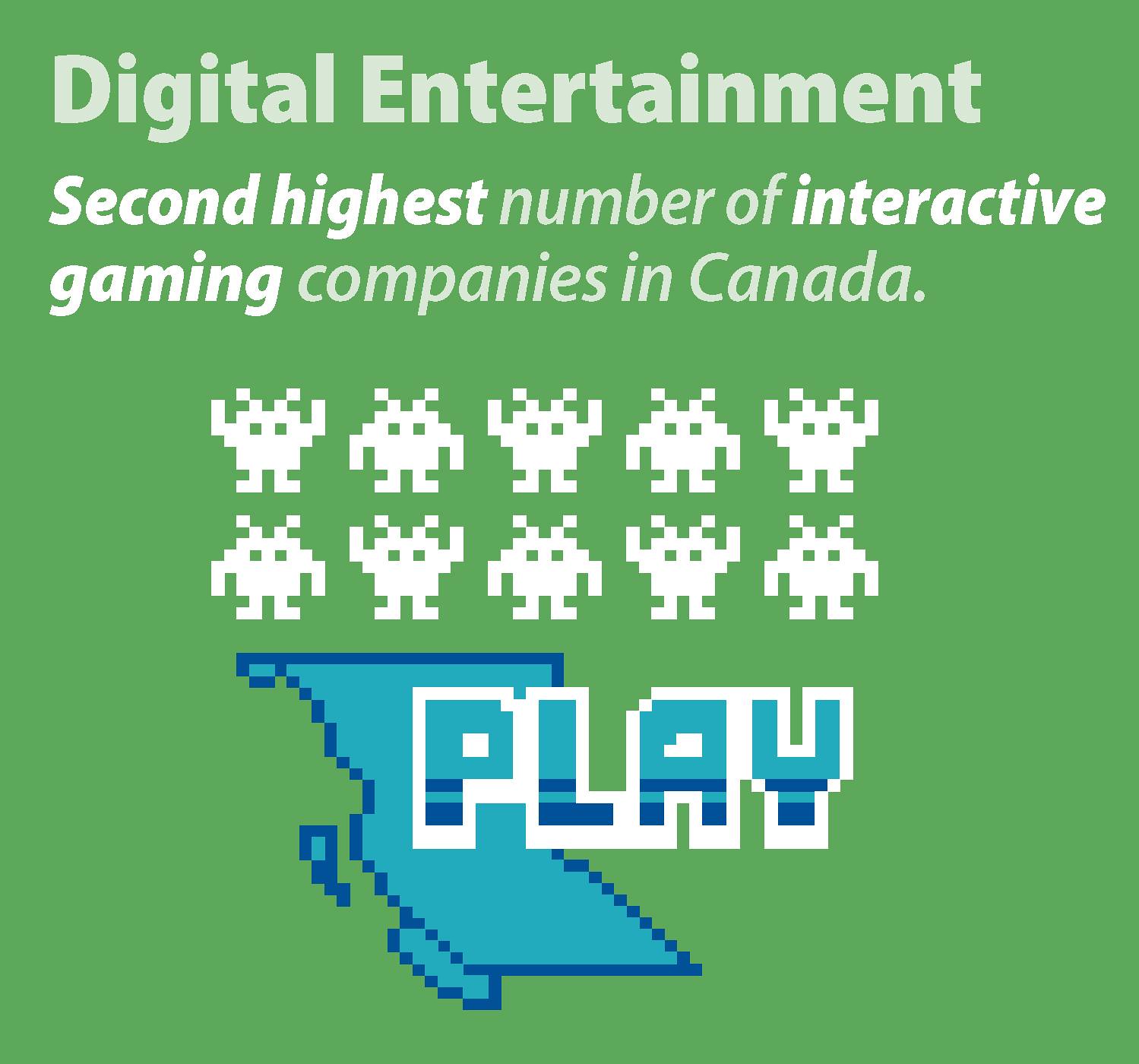The image features a digital display on a green background. At the top, in light blue letters, it reads "Digital Entertainment." Beneath this, in italicized white text, it states, "second highest number of interactive gaming companies in Canada." Below the text, there are two rows of pixelated characters, reminiscent of creatures from an early 1980s video game like Space Invaders. Each row contains five creatures with antennae, alternating their positions up and down. Directly under the rows of characters, the word "play" is prominently displayed in blue letters. Behind this word, a subtle, diagonally placed outline of the province of British Columbia can be seen, light blue with a dark blue border, further enhancing the retro, 8-bit aesthetic of the image.